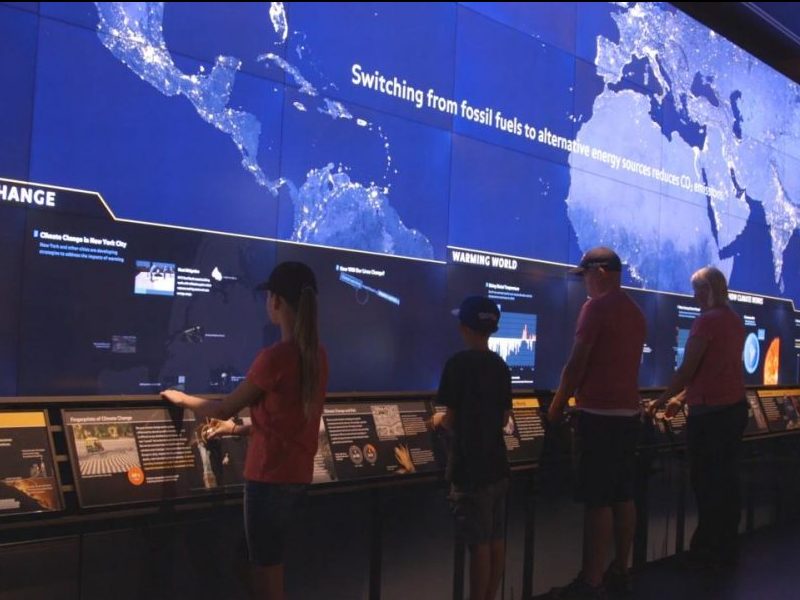The image depicts a museum exhibit focused on climate change and alternative energy sources. The exhibit features a massive, wall-sized screen displaying a satellite image of the Earth, highlighting various regions including Central America, the Caribbean, South America, Europe, the Middle East, and northern Africa. The continents are portrayed in light blue, while the oceans are depicted in dark blue. Prominently placed text across the screen reads, "Switching from fossil fuels to alternative energy sources reduces CO2 emissions." Below this, a smaller screen provides additional information on climate change and global warming.

In front of this impressive display, four individuals are engaged with interactive kiosks that offer detailed presentations on the subject matter. Among the visitors are a family consisting of two parents and their children. Both parents and children have baseball caps. The daughter, who is blonde and wearing a pink shirt, is interacting with one of the screens, while the son, dressed in a black shirt and cap, is at another kiosk. The father, also wearing a cap and dressed in a pink shirt and shorts, stands next to the son. The mother, likewise blonde and in a pink shirt, is close by. The scene captures the educational and interactive nature of the exhibit designed to inform and engage visitors on the importance of transitioning to alternative energy to combat climate change.